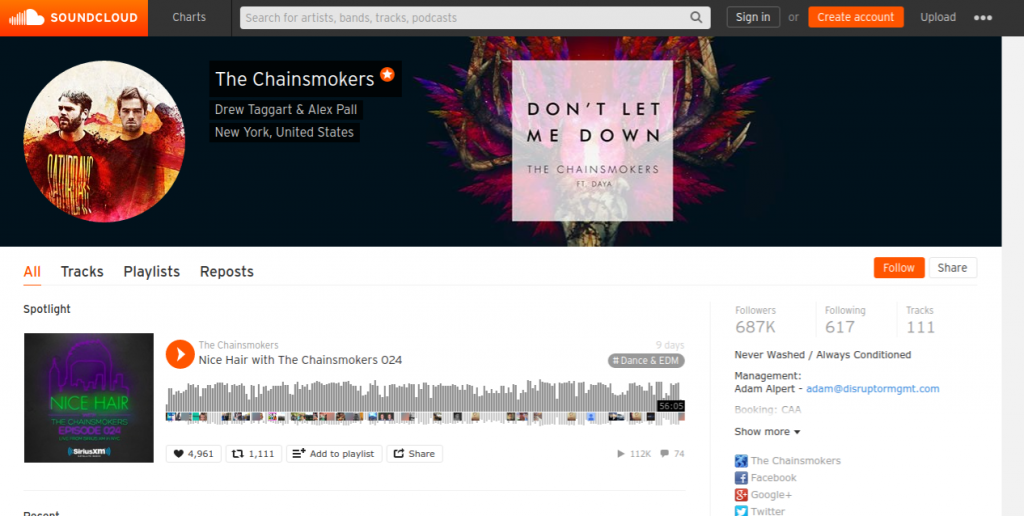This image captures the SoundCloud profile for The Chainsmokers, a music duo consisting of Drew Taggart and Alex Pall from New York, United States. The top section of the website features a black header. Within this header, there is an image of a vinyl record displaying a photo of The Chainsmokers. In the picture, both members are sporting dark and light red shirts against a white background. The shirts feature yellow lettering that spells out "Chainsmokers."

Within the black header, there's also a smaller white box in the center, which highlights the album name "Don't Let Me Down" by The Chainsmokers. This album is noted as having a number one song. On the same SoundCloud page, users are given the option to play a snippet of their song titled "Nice Hair with The Chainsmokers."

The top left corner of the SoundCloud website prominently displays the word "SoundCloud" in white font against an eye-catching orange background. Next to the SoundCloud logo, there are additional options including "Charts," a search function, "Sign In," "Create Account," and "Upload," all conveniently positioned for easy navigation.